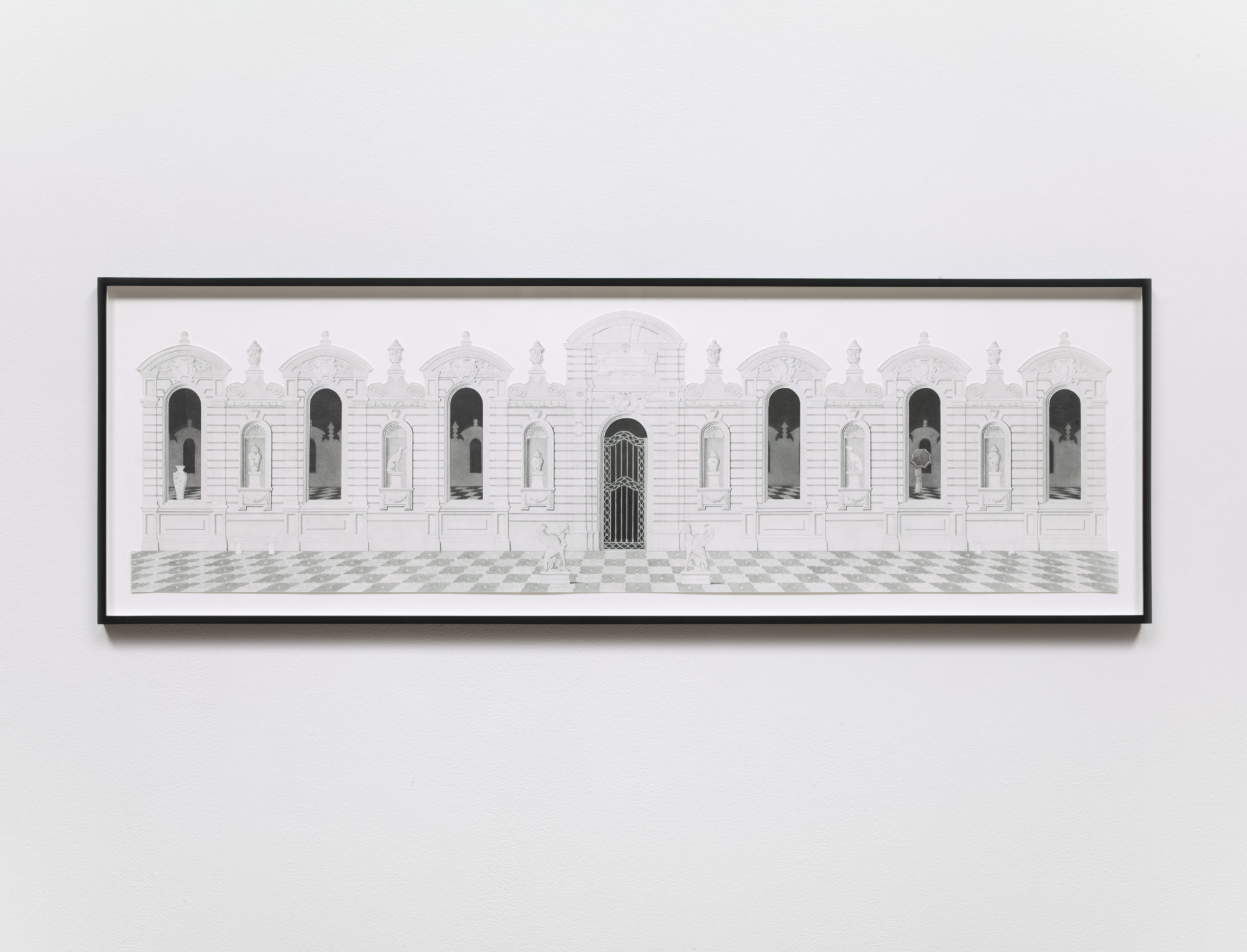The image depicts a very long rectangular picture hanging on a light gray wall, encased in a slim black frame. The central subject of the image is a striking white building with a symmetrical façade. This building features six distinct arched windows—three on the left and three on the right—each containing various gray silhouettes of different shapes visible through the glass. Centrally placed is a gray, metal barred doorway capped with a large rounded arch. Flanking the door and windows are spikes that point upwards; some of these are level with the roof, while others sit atop smaller arches. In the foreground, a gray and white checkerboard design stretches out on the floor, enhancing the building's stately appearance. The entire scene appears against a white background, amplifying the building's prominent white structure and intricate features.